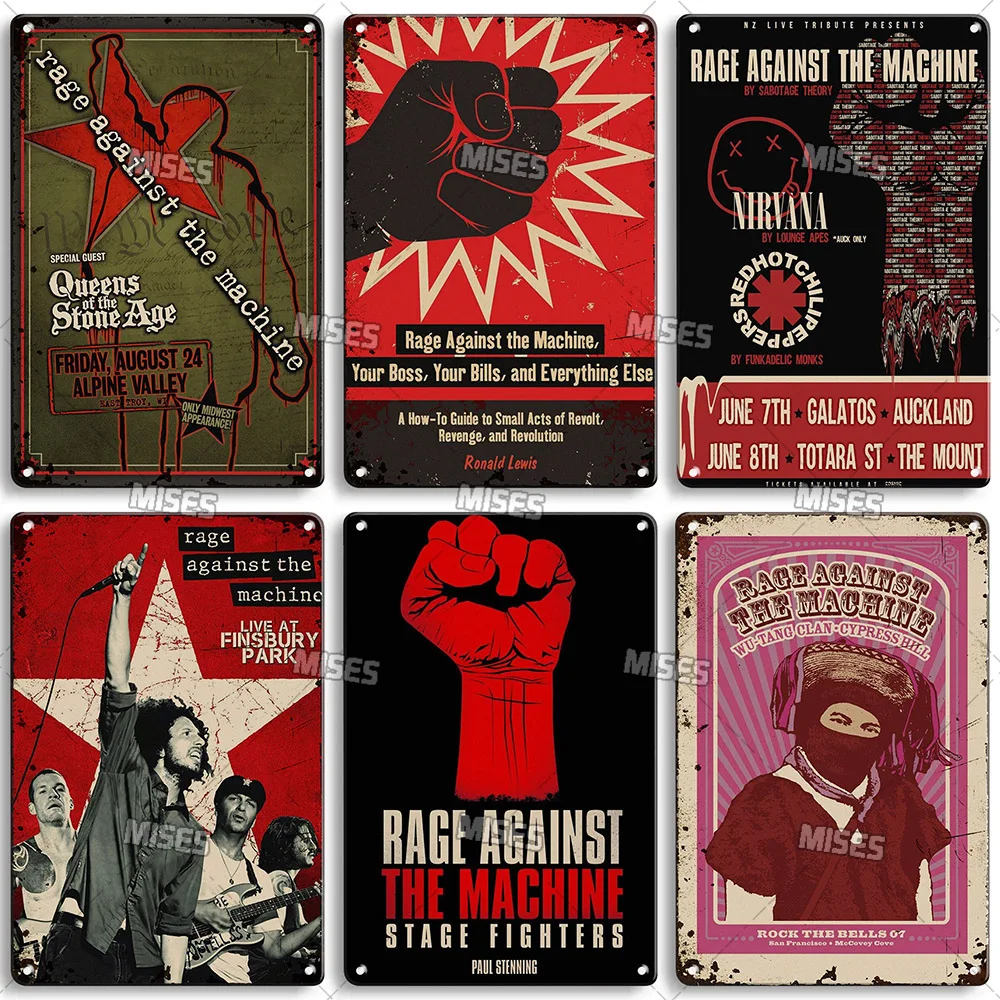The image is a detailed collage of six concert posters predominantly featuring the band Rage Against the Machine. Starting from the top left, the first poster is a primarily olive green design showcasing an outline of a body with a raised fist and a red star, prominently branded with 'Rage Against the Machine' and details about a concert featuring special guests Queens of the Stone Age, scheduled for Friday, August 24th, at Alpine Valley. To its right, the second poster, rendered in red, frames a black fist with the bold proclamation 'Rage Against the Machine, Your Boss, Your Bills, and Everything Else,' emphasizing themes of revolt and revolution. 

The third poster within the top row is mainly black, inscribed with 'Rage Against the Machine' diagonally and subtitled 'Sabotage Theory'. Below these, the bottom row begins with a predominantly red and white collage featuring the band members' faces and star iconography, captioned 'Rage Against the Machine, Live at Finsbury Park'. The next poster, striking with a red fist against a black background, declares 'Rage Against the Machine, Stage Fighters.' 

Finally, the sixth poster, with tones of pink, black, and white, portrays a person in a face mask and marks a collaborative event listing 'Rage Against the Machine, Wu-Tang Clan, Cypress Hill'. The posters within this collage are artistically varied yet unified by their militant and rebellious iconography and themes, depicting a blend of concert announcements and revolutionary sentiment.